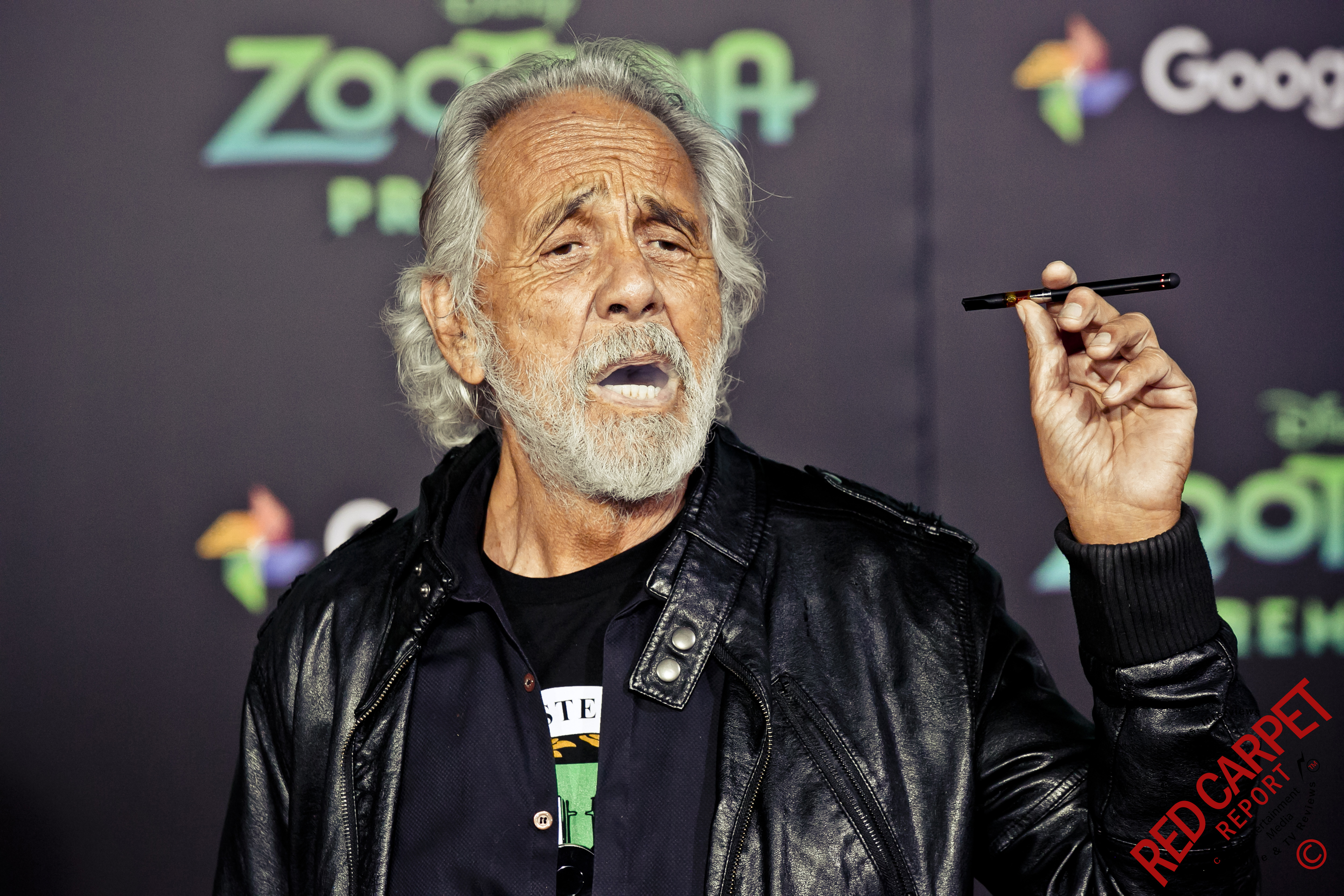The image features Tommy Chong standing in front of a black backdrop at the Zootopia premiere, as inferred from the visible Zootopia logo and Google logos behind him. Chong, who has wavy, chin-length gray hair and a full white beard, is dressed in a layered outfit consisting of a black leather jacket, a navy blue button-up shirt, and a black t-shirt beneath that. His left hand is raised, holding a black pen, while his facial expression suggests mock sadness, with his eyebrows furrowed together. The bottom right corner of the image shows the red text "Red Carpet Report" along with a copyright symbol.